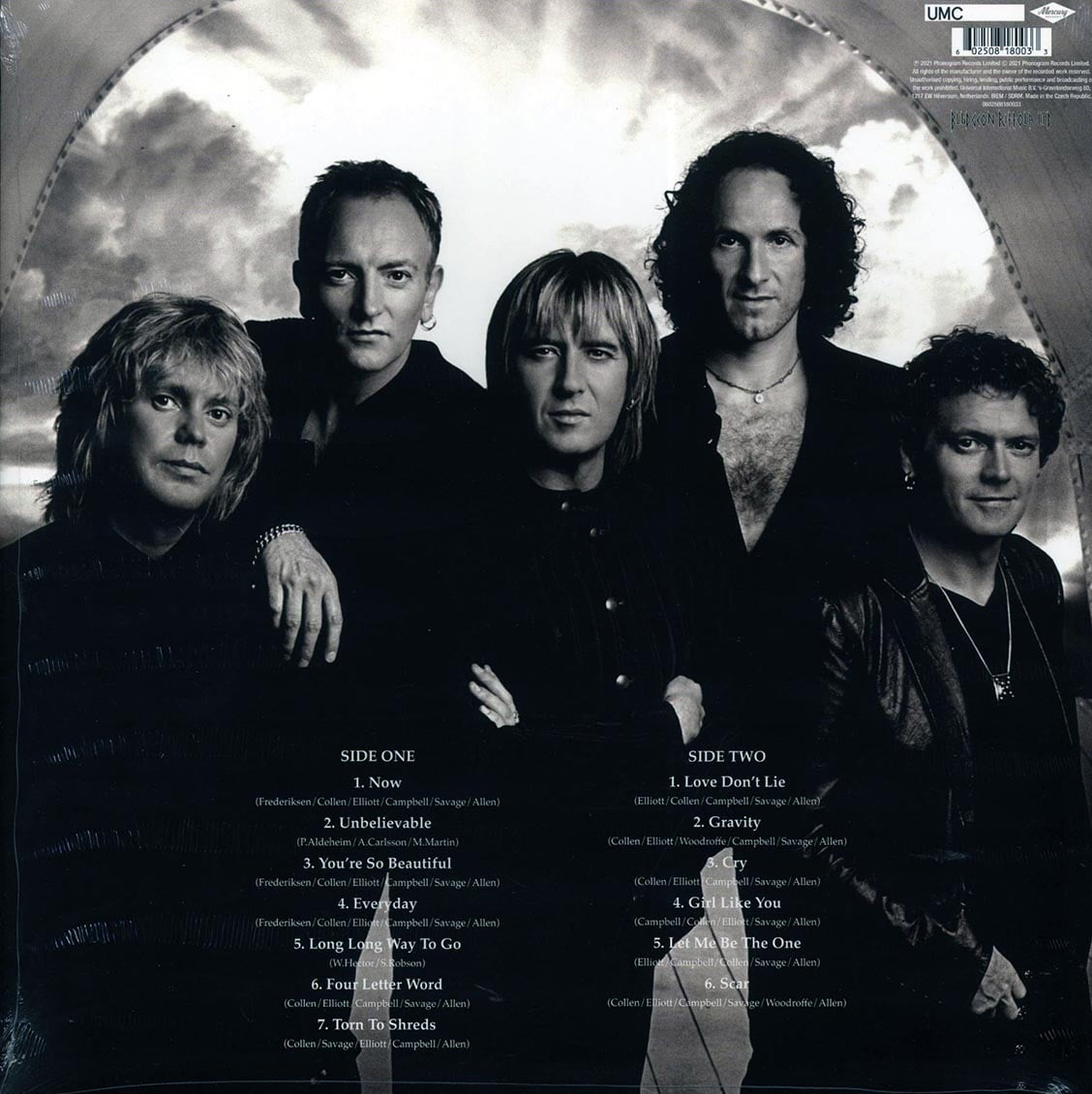The image appears to be the back cover of a black-and-white album or CD, featuring five men, likely the artists, who are positioned in various poses with some having their arms crossed or around each other, and they're smirking into the camera. Their attire is predominantly black, with some wearing funky clothing and jewelry, including earrings and necklaces. Four of them have long hair, while one distinctively has short hair and a leather coat. The group is standing in a tunnel-like setting with light visible behind them and curved walls surrounding them. At the bottom of the cover, song titles for side one and side two are listed in white font. Side one includes tracks like "Now," "Unbelievable," "You're So Beautiful," "Every Day," "Long Long Way to Go," "Four Letter Word," and "Torn to Shreds." Side two comprises "Love Don't Lie," "Gravity," "Cry," "Girl Like You," "Let Me Be the One," and "Scar." In the upper right corner, small print information is present, including a white box with "UMC" and a UPC code.